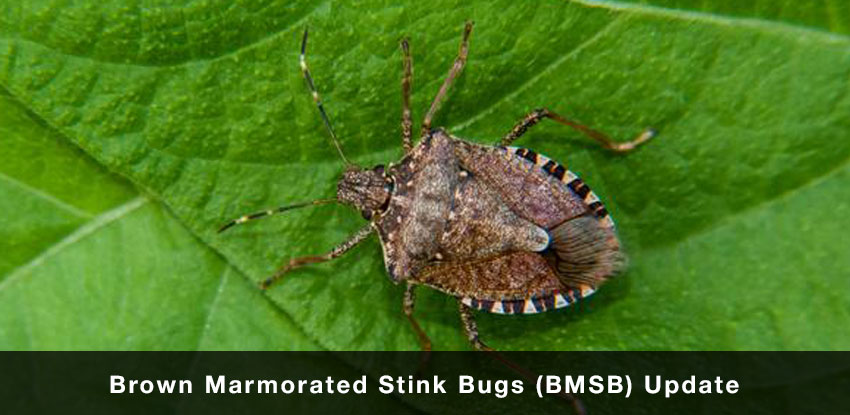The photograph features a detailed and centered image of a brown marmorated stink bug (BMSB) perched on a vibrant, well-hydrated green leaf, which contrasts nicely against the bug's brown and patterned body. The stink bug, resembling a shield in shape, occupies the majority of the rectangular frame with its head facing the upper left corner. Its distinctive shell is marked with black and slightly orange patterns, and has a unique, jutting component that sets it apart from the rest of its exoskeleton. The legs and shiny, gold-colored antennae splay outwards in typical insect fashion. The image also captures intricate details like the leaf's veins and the stems in the background. Beneath the photograph, there is a black banner with white text, stating "Brown Marmorated Stink Bugs (BMSB) Update," providing context and identification for the viewer.